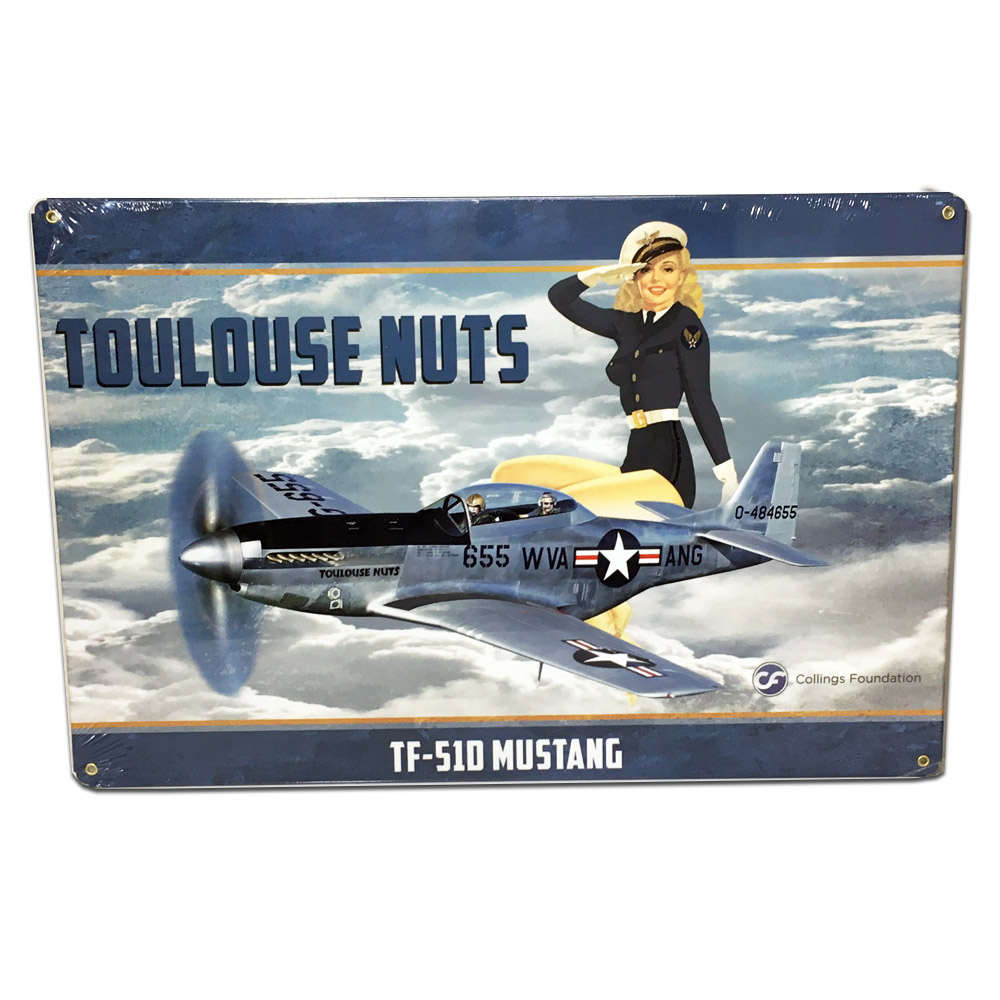The image is an advertisement depicted on what appears to be an old metal sign. It prominently features a World War II-era fighter jet labeled "TF-510 Mustang," which is sleek and silver with one propeller, and also bears the inscriptions "655 WVA ANG" and "0-484-655" on its tail. In bold blue letters, the top section of the advertisement reads "Toulouse Nuts," a playful name presumably inspired by the city of Toulouse. The sky-blue background adorned with gray-white clouds frames a visually striking illustration of a blond pin-up girl dressed in an American Air Force uniform, complete with short shorts, white gloves, and a white hat. Saluting and sitting atop the airplane, the woman serves as the central focus of the sign, adding a nostalgic and patriotic flair to the overall design. Additionally, there is a note of accreditation to the "CF Collings Foundation" in the lower right-hand corner.